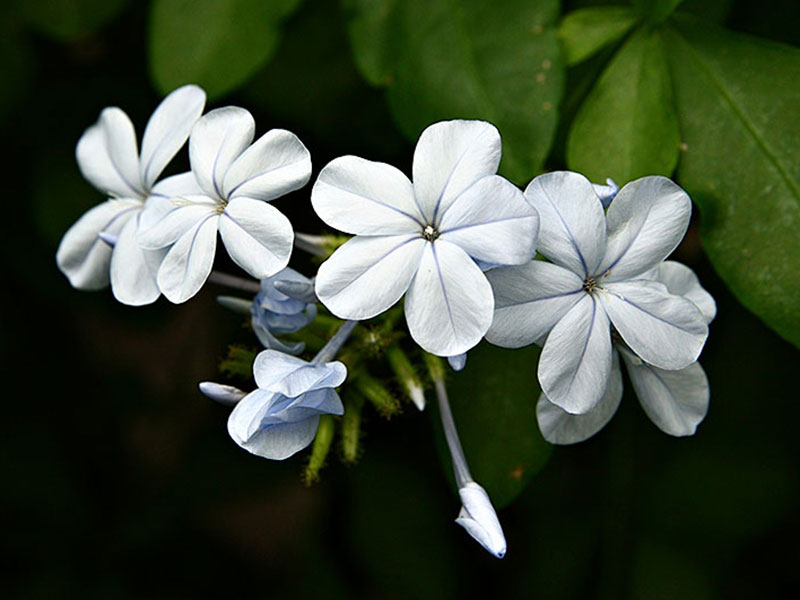This image showcases a cluster of white flowers set against a dark background, suggesting it was taken in early spring. The flowers, which are centrally positioned, display varying states of bloom; five to six are fully open, revealing rounded petals with a distinct black vein down the center, while about four are still in the process of opening. One flower is captured midway through its bloom, adding dynamic interest to the composition. In the backdrop, the dark space punctuates the lush greenery and leaves that feature prominently, enhancing the contrast. Additionally, a single blue flower is discreetly nestled amongst the white blooms, visible around the left-center region of the picture. Stems and buds cascade from the upper center towards the lower center, creating a harmonious balance of elements. The intricate detail in the petals and leaves further suggests that this image may be a drawing or painting rather than a photograph.